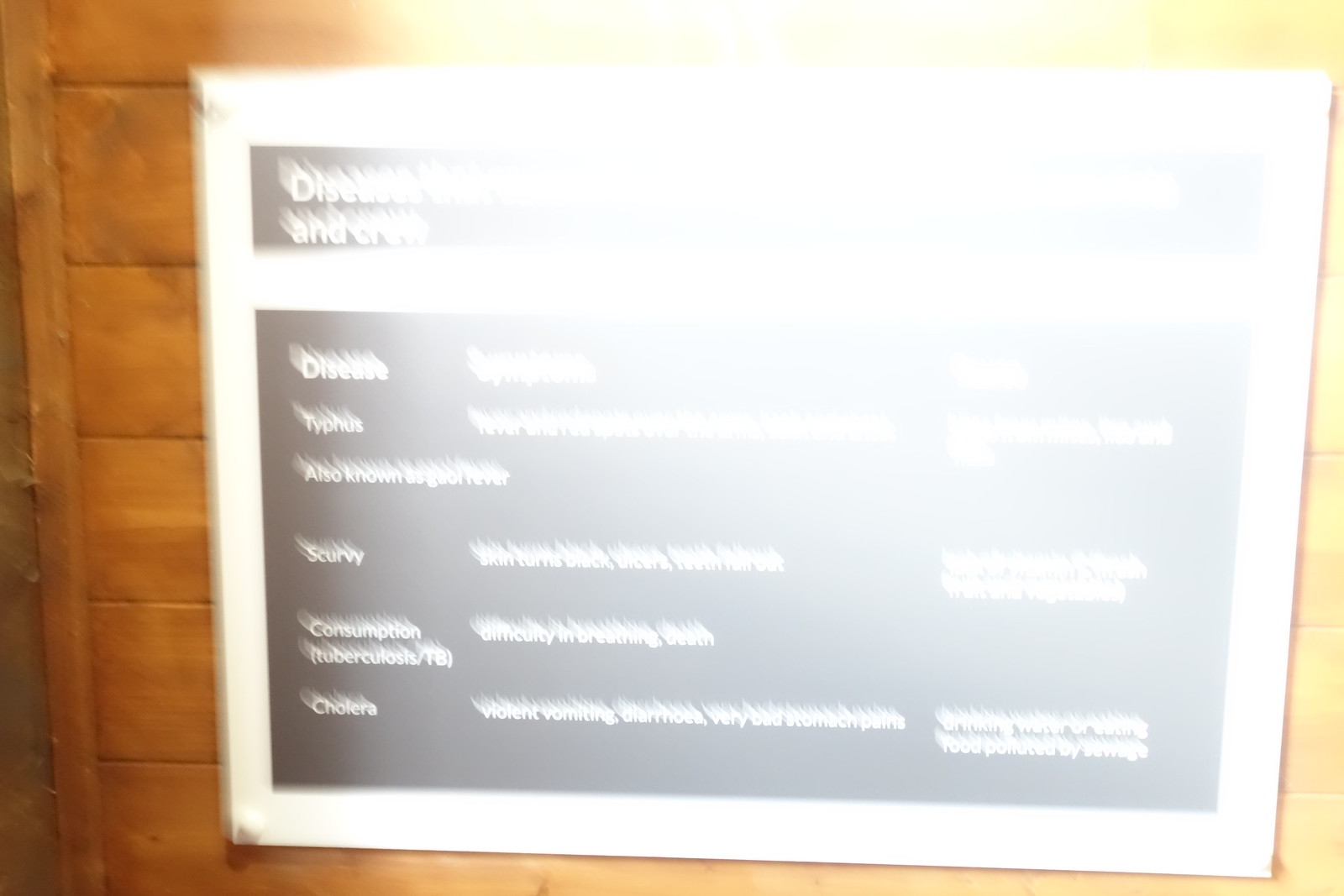This photograph captures an up-close, very blurry image of a sign hanging on a horizontally planked wooden wall, which is an orange, reddish-brown color. The right three-quarters of the photo is illuminated by a light, casting a yellow tint over that section of the wall, while the left edge reveals the true color of the wood. The sign itself is primarily a large white square featuring an upper black rectangle with two lines of unreadable white text. Below that, an even larger black rectangle occupies most of the bottom portion of the sign, containing several rows of similarly indistinct white writing arranged in six lines across three columns. The center of the photo is notably faded and turns white, possibly due to overexposure from the camera flash, further obscuring the details.